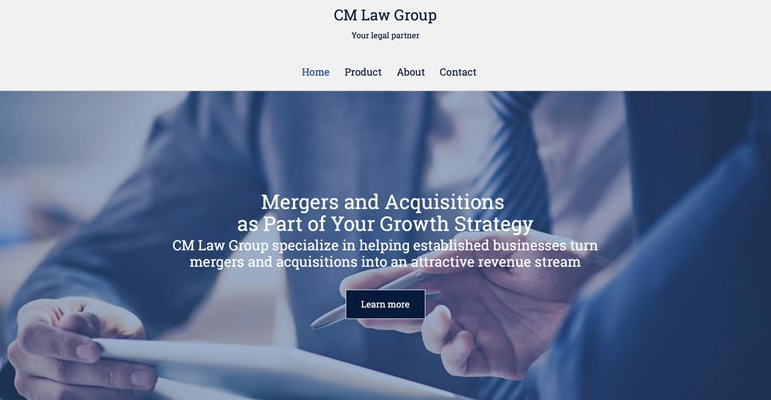This is a detailed and cleaned-up version of the caption:

---

The opening page of the CM Law Group website prominently features a professional image that captures the essence of their services. Central to the image is a person wearing a dark suit, white dress shirt, and a tie, holding a tablet. The individual’s head is not visible, emphasizing the professionalism and focus on the service rather than the person. Standing to the left of this individual (from the viewer's perspective) is another person, extending their right hand with a pen, suggesting a moment of agreement or contract signing.

At the very top of the webpage, the navigation bar displays the options: "Home," "Product," "About," and "Contact," under the bold heading "CM Law Group - Your Legal Partner."

In the center of the image, white text reads: "Mergers and Acquisitions as Part of Your Growth Strategy. CM Law Group specializes in helping established businesses turn mergers and acquisitions into an attractive revenue stream." This text integrates seamlessly with the visual elements of the image, maintaining a professional and cohesive appearance.

Below this central text, there is a dark, clickable box inviting visitors to "Learn More," providing a clear call-to-action for potential clients seeking further information about the firm’s services.